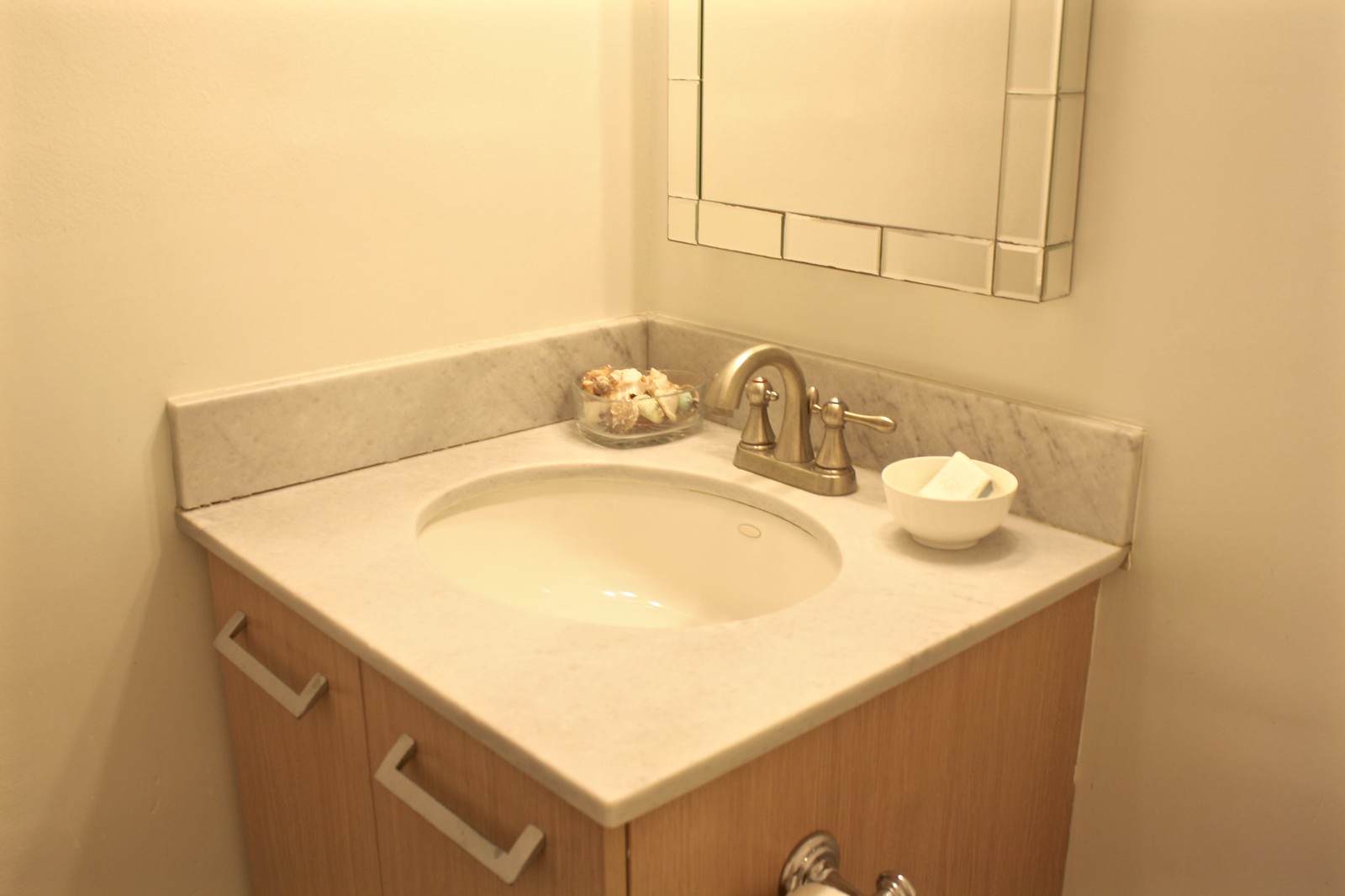This photograph showcases a pristine, all-white bathroom interior, focusing on the corner where the left and right walls meet. Dominating this corner, we find a sleek white sink basin. The right wall above the sink features a partially visible mirror with a silver border, intricately lined to create a rectangular yet square-like shape. Although only the lower half is in frame, its elegant design is evident. 

Directly above the sink, a marble splash guard provides both functionality and a touch of luxury. The sink is equipped with a polished silver faucet and matching handles. To the right of the faucet, a white bowl holds a white square object, possibly a soap dish or a decorative item. On the left side, a charming faux plant in a small dish adds a hint of greenery and liveliness to the monochromatic scene.

Beneath the basin, two cabinet doors, each adorned with silver handles, offer storage and complete the minimalist yet sophisticated look of this immaculate bathroom corner.